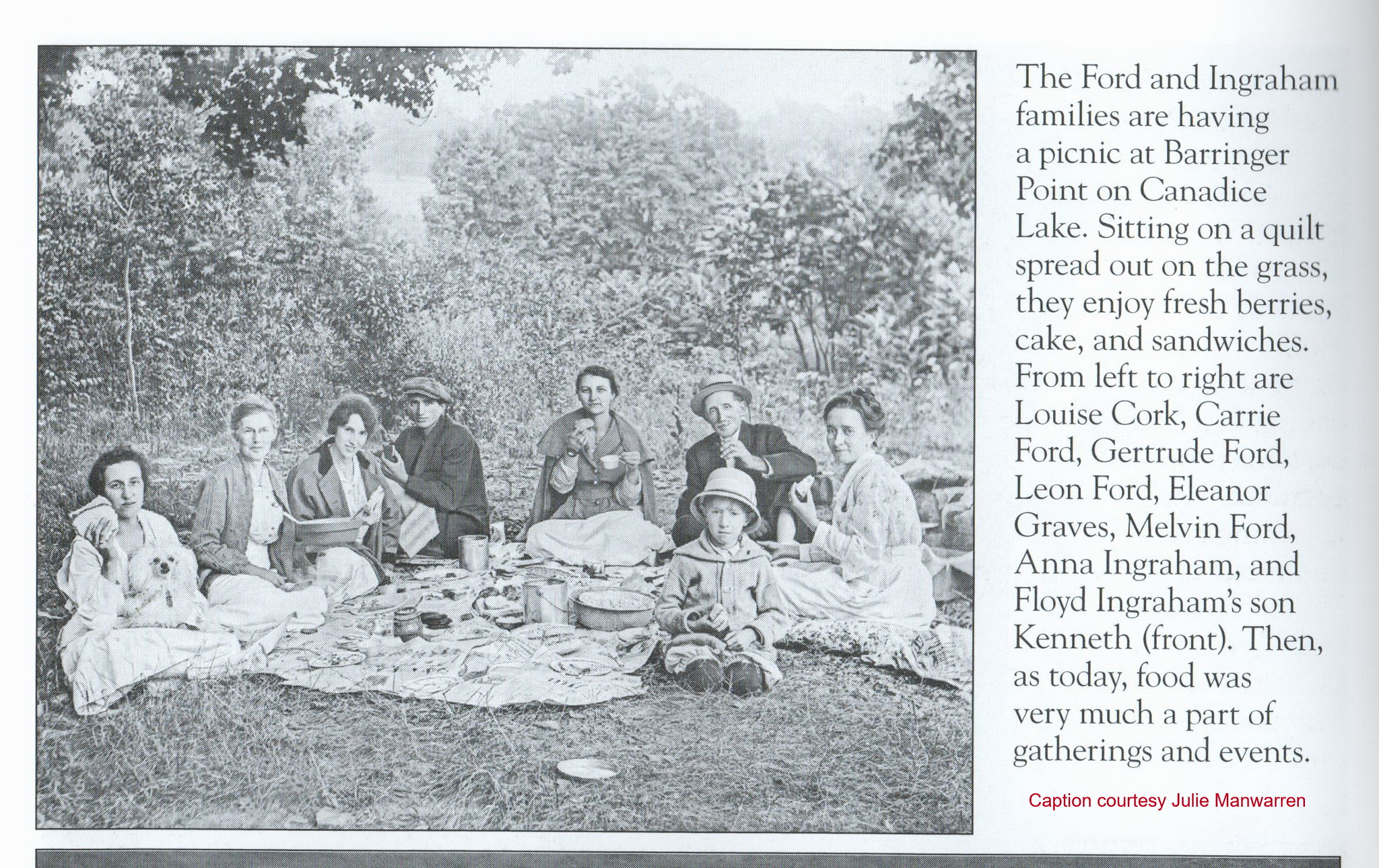The black and white photograph captures a vintage picnic scene, likely from the early 1900s, set in a forest clearing at Barringer Point on Cannadice Lake. The image features eight individuals, including seven adults and one child, who are members of the Ford and Ingraham families. They are seated on a quilt spread out on the grass, around which a variety of picnic items like bowls, pots, cups, fresh berries, cake, and sandwiches are arranged. The serene backdrop of trees frames this gathering. From left to right, the attendees are identified as Louise Cork, who has a dog in her lap, Carrie Ford, Gertrude Ford, Leon Ford, Eleanor Graves, Melvin Ford, Anna Ingraham, and in the front, Floyd Ingraham's son Kenneth. This nostalgic image, captioned courtesy of Julie Mann-Warren, highlights the timeless tradition of sharing food during family gatherings and events.